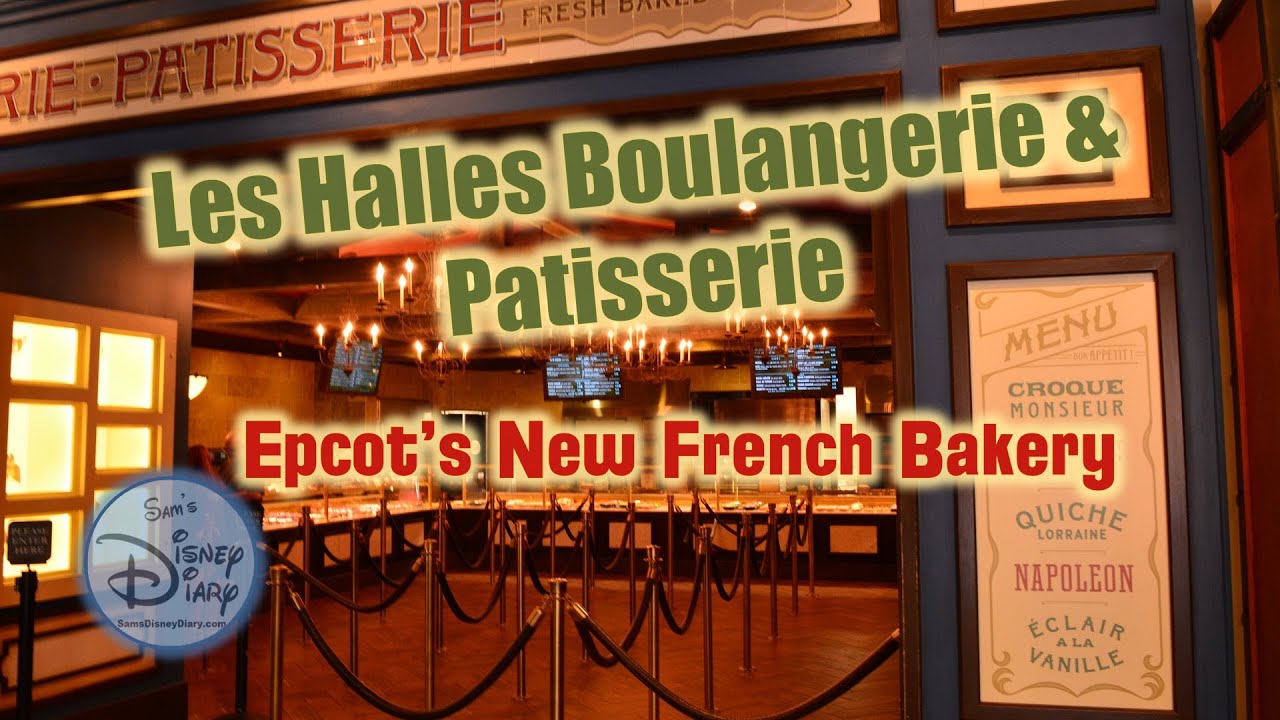This detailed advertisement poster for Epcot’s new French bakery, titled "Les Halles Boulangerie & Patisserie," showcases a well-lit shop interior, possibly situated within a mall. A prominent, open doorway displays a large sign reading "Patisserie Fresh Bake," welcoming visitors into the roped-off area aimed at managing customer flow. Against a dark blue wall to the right of the entryway is a framed menu listing items like Croque Monsieur, Quiche Lorraine, Napoleon, and Éclair à la Vanille. Across the top of the image, the bakery's name is prominently displayed in green font outlined in yellow, while beneath it, in red font with the same yellow outline, it reads "Epcot's New French Bakery." The bottom-left corner is marked with a Disney logo and the text "Sam's Disney Diary." The polished setting and clear signage, including chandeliers and neatly arranged tables along the edges, complete this inviting and informative visual.